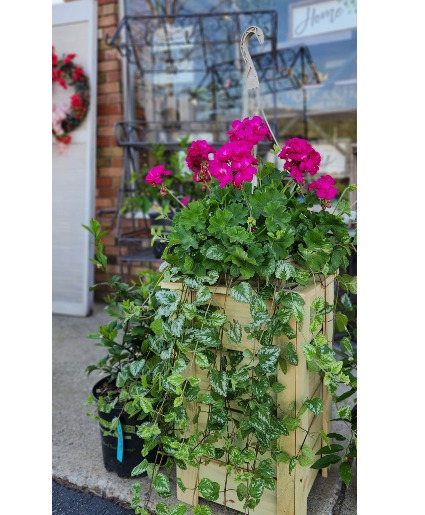The photograph depicts the exterior of what appears to be a floral shop, identifiable by a wreath adorned with red flowers hanging on a dark-colored door in the background. Central to the image is a tall, beige, wooden structure housing an abundance of green leaves and vibrant magenta flowers extending downward and seemingly overflowing its confines. To the left of this structure, there is a black flower pot on the ground, partially obscured by the sprawling leaves from the wooden enclosure. The background features a dark red-brown brick wall and a window displaying a sign with the word "home." Various metal objects are visible near the window, enhancing the rustic outdoor setting.